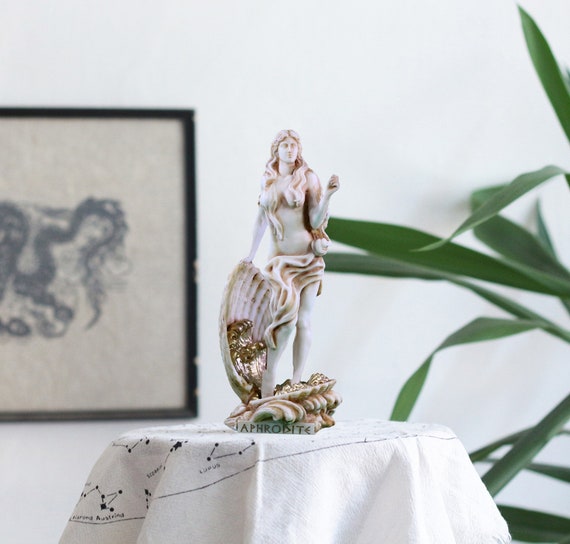This detailed image depicts a small, intricately crafted statue of Aphrodite, positioned on a round, cloth-covered table. The base of the statue bears the inscription "Aphrodite." The statue, primarily white—possibly made of marble or ceramic—features Aphrodite emerging from an open seashell. Her long hair cascades down, covering her chest, and a cloth is draped around her hips. She holds onto the shell, which appears to contain a gold-colored object or adornment. Surrounding the base are additional smaller shells. The backdrop includes a white wall, a black-framed painting to the left, and green leaves from a houseplant on the right, indicating the setting might be an indoor space such as a home or an art gallery. Additionally, the tablecloth under the statue features a pattern of black lines and dots, possibly representing constellations. The visual elements suggest a theme melding classical art with subtle astronomical motifs.